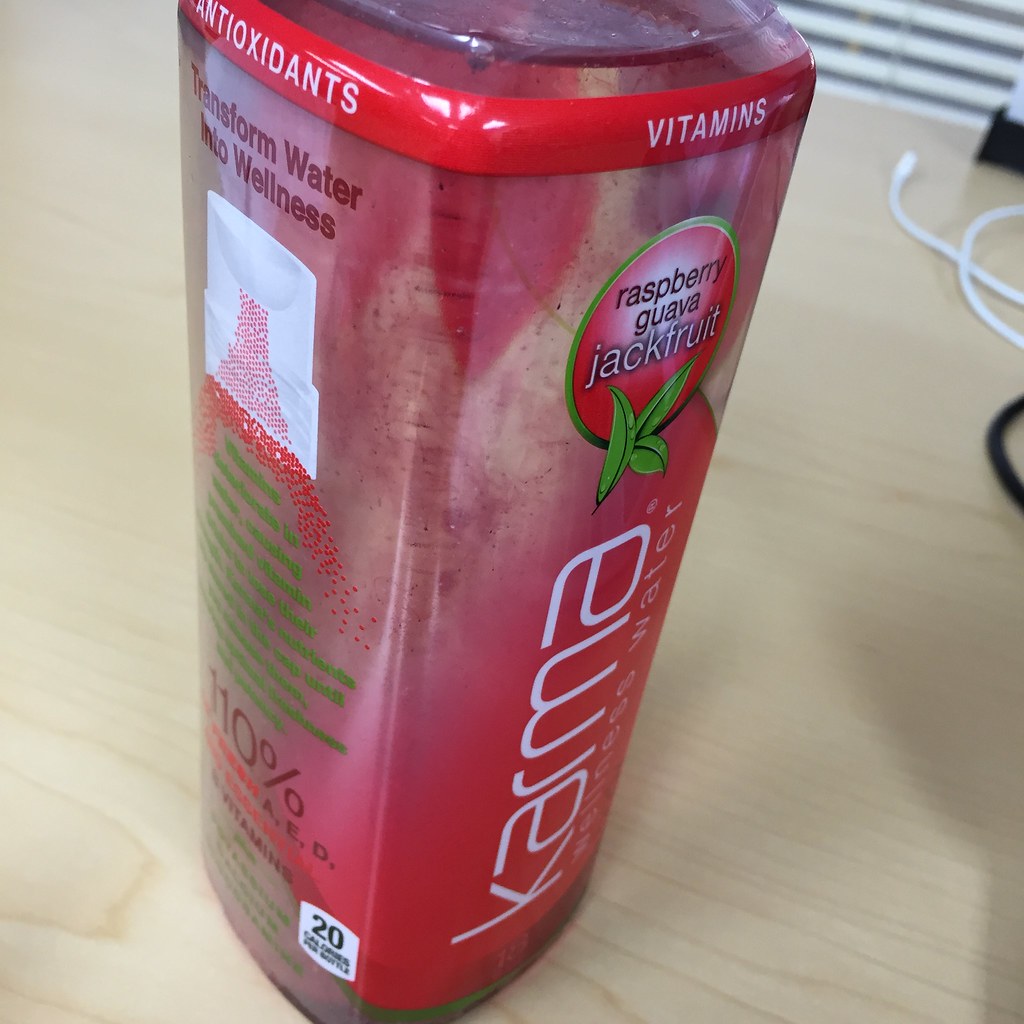This close-up image captures a bottle of Karma Wellness Water, prominently showcasing its raspberry guava jackfruit flavor. The bottle is rectangular with a reddish berry-colored label, featuring white text and some green highlights. Key phrases include "antioxidants," "vitamins," and "transform water into wellness." Although the detailed text on the side is not readable due to the angle, the partial numbers "110%" and "20," potentially indicating nutritional values or calories, are visible. The bottle appears almost empty. It rests on a light beige woodgrain table, and various background elements such as white window blinds and a few stray cords, including a phone charger, are slightly out of focus off to the right.